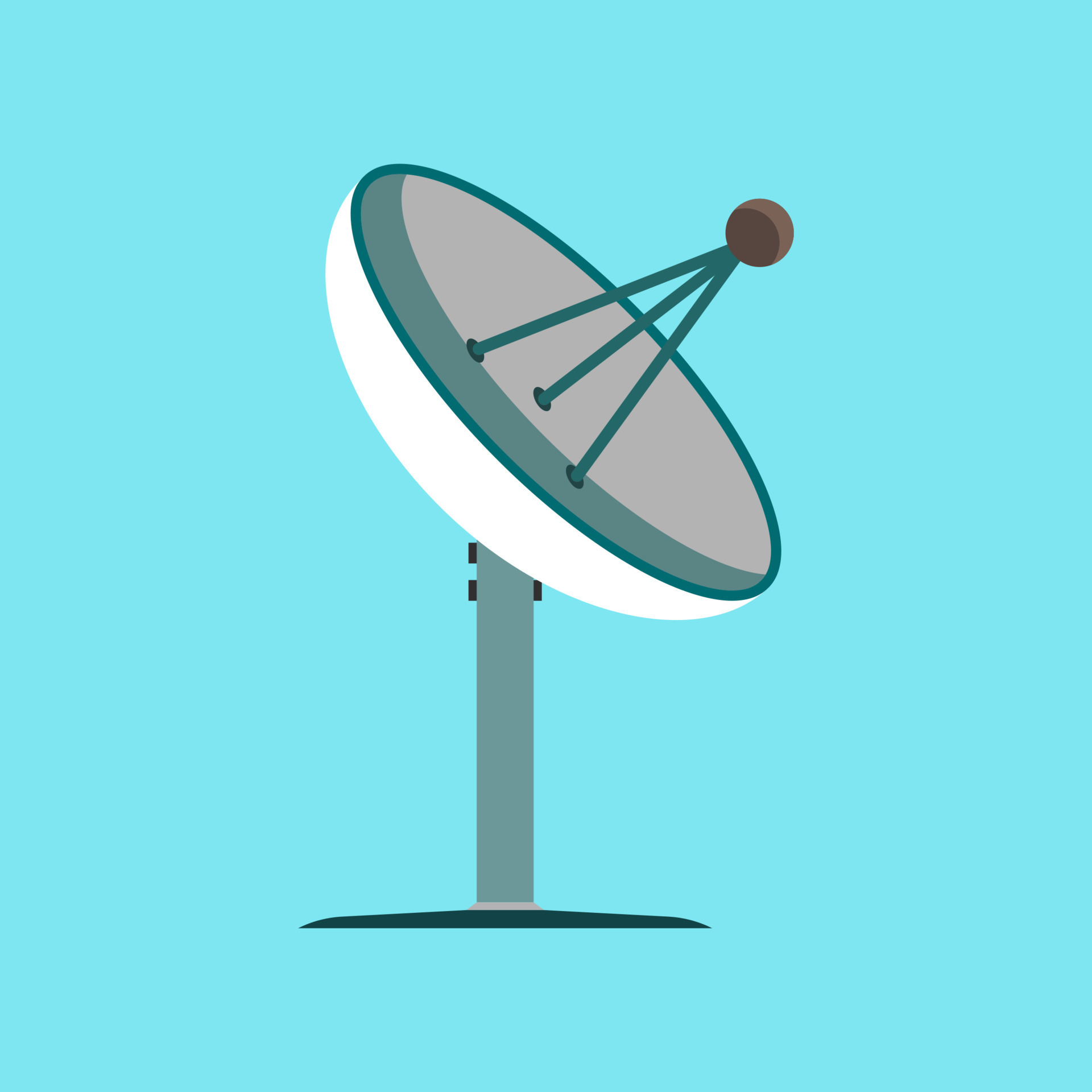This image features a simplistic, two-dimensional, cartoon-style drawing of a satellite dish set against a light teal or turquoise background. The base of the dish is black or dark gray, leading up to a gray pole that supports the white satellite dish itself. The dish attaches to the pole via black clamps. The central part of the dish includes a brown or red cone-like antenna, which is connected by three grayish supports extending from the dish. The drawing has no text and is stylized without any shading or texture, making it look like clip art or a computer-generated image, suitable for use on websites or as an icon to denote a satellite dish. The dish points towards the top right of the image, and the entire illustration maintains a simple and flat visual style.